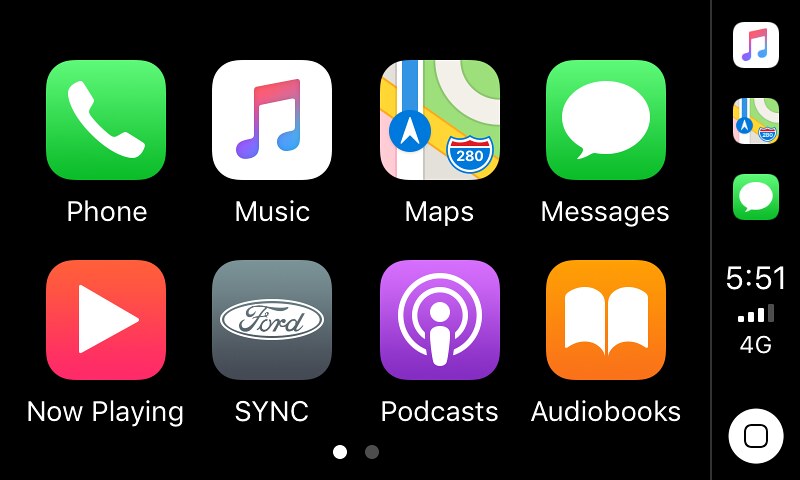This close-up image depicts the screen of a smartphone after it has been turned on, showcasing a variety of app icons neatly arranged in a grid layout against a black background. Each app icon is square-shaped with rounded corners, adhering to common smartphone design aesthetics.

Prominently, the first row of icons features a green app with a white telephone symbol, labeled 'Phone'. Next to it is a white app featuring pink and blue music notes, set against a purple background, identified as a music player. The third icon in the sequence is an app named 'Maps', characterized by a blue, yellow, and green design and marked with a red and blue depiction of Highway 280. Completing the row is a green app depicting a white speech bubble, named 'Messages'.

In the second row, starting from the bottom, the first icon is red with a white triangle, labeled 'Now Playing'. Adjacent to it is a gray app featuring the white Ford emblem, named 'Sync'. Further along is a purple app displaying a white figure with rings around it, identified as 'Podcast'. Finally, an orange app with the image of two opened book pages in white is labeled 'Audiobooks'.

Additionally, on the right side of the screen, there appears to be a vertical toolbar displaying various indicators: it is 5:51 PM, the device has 4G connectivity. The side also features icons for music, maps, and messages, as well as a white circle with a black app inside it.